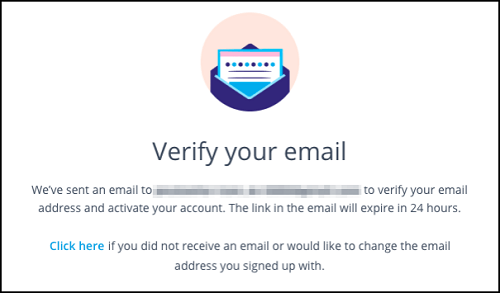This image is a detailed screenshot of a "Verify Your Email" pop-up. The pop-up is a squarish rectangle, outlined with a thin black line. The interior is white. At the top center, there's a peach-colored circle containing a blue envelope with a blue letter emerging from it. The top of the letter features a white rectangle with a pink banner across the top. Below the banner are alternating navy blue and bright blue dots, followed by two blue lines.

Directly beneath the envelope illustration, in bold black text, it reads, "Verify Your Email." This is followed by smaller black text stating, "We've sent an email to," with the email address blocked out for privacy. The message continues, "To verify your email address and activate your account, click the link in the email. The link will expire in 24 hours."

After a small gap, there's blue text that reads, "Click here," followed by black text indicating, "if you did not receive an email or would like to change the email address you signed up with..."